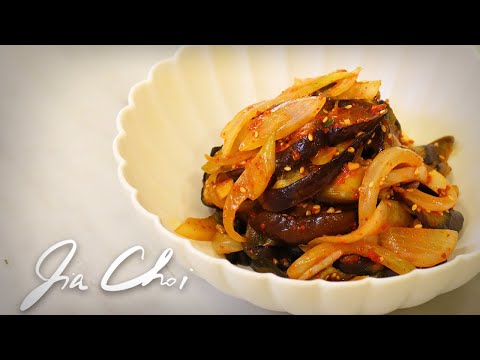This image features a slightly wider-than-tall perspective, framed by black letterboxed areas at the top and bottom, constituting about 10-15% of the total frame. The primary focus is the central area with an off-white (cream-colored) background, resembling a tabletop surface. Dominating the right side of the image, an off-white scalloped bowl occupies approximately two-thirds of the width.

In the lower left corner of the image, there is a signature in white cursive text that appears to read "J-A C-H-O-I," though the exact letters are somewhat unclear. The bowl itself is elegant with its scalloped edges and contains a visually appealing dish. It appears to be composed of moist noodles and meat, possibly mixed with a savory sauce. Among the ingredients, there are hints of sautéed onions, along with possible slices of eggplant or zucchini. The dish is garnished with sesame seeds and a scattering of red pepper gochugaru flakes, suggesting a fusion of flavors potentially inspired by Asian cuisine. The presentation is careful, with no smudges on the edges of the bowl, emphasizing a tidy and appetizing arrangement.